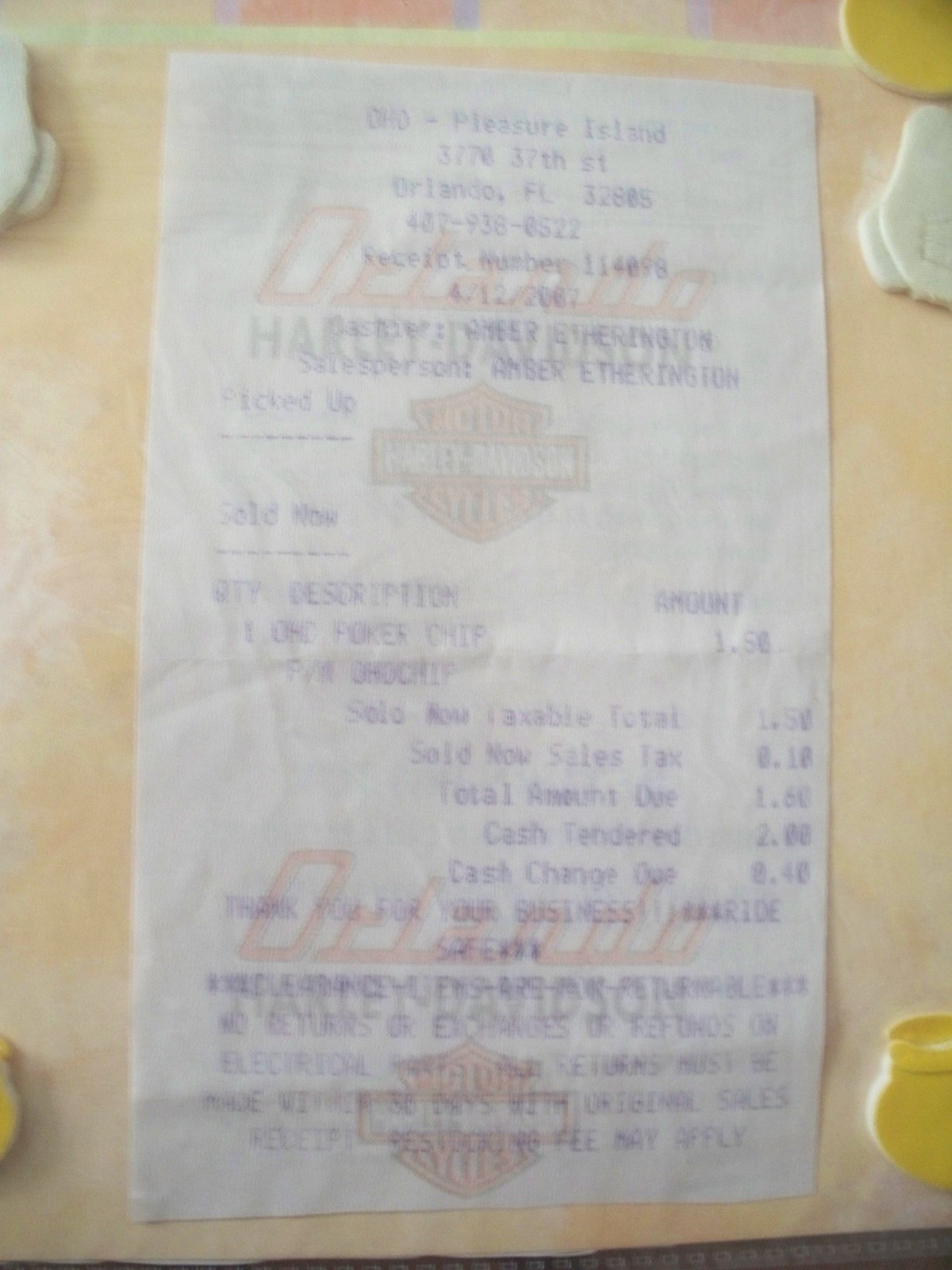A somewhat blurry photograph captures a receipt laid on a tan counter or surface. The receipt is printed in blue ink atop a faint background logo of the establishment. The heading features "Orlando" in a stylized, curvaceous font, followed by a Harley-Davidson logo. The receipt details the address: Pleasure Island, 3770 37th Street, Orlando, Florida, 32805, with the contact number 407-938-0822. The lower section, though challenging to read, includes the sales representative's name, likely Amber Etherington. The recorded transaction indicates a purchase amounting to approximately $2 or $1.60.